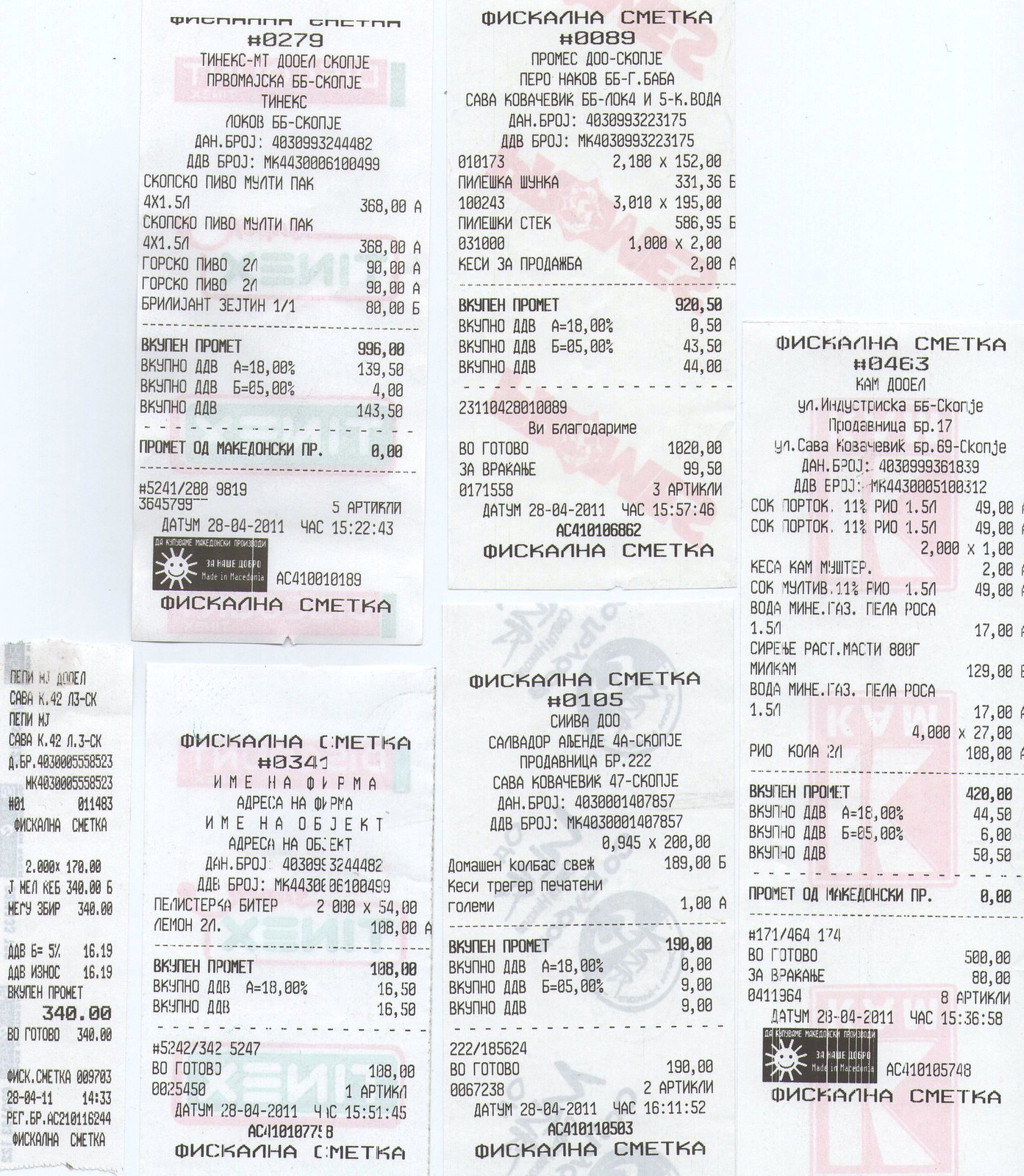In this color portrait-format photograph, there are six receipts arranged with two on top and four on the bottom. Each receipt is white with predominantly black text, accented by vibrant red logos, though one features a black logo. These repetitive logos and consistent watermark patterns suggest they are all from the same company. The text on these receipts includes both numbers and letters, with a prominent line in bold at the top reading "H C K A N H A C M E T K A." The script uses characters that look similar to English letters, though the language appears to be an unfamiliar, possibly Eastern European, language. Prices and quantities are also listed in this foreign script and currency. Two receipts—one in the upper left and one on the bottom right—stand out by having a black area with a sunshine emblem. The overall image has a slight red tint, adding to the uniform appearance of the receipts.